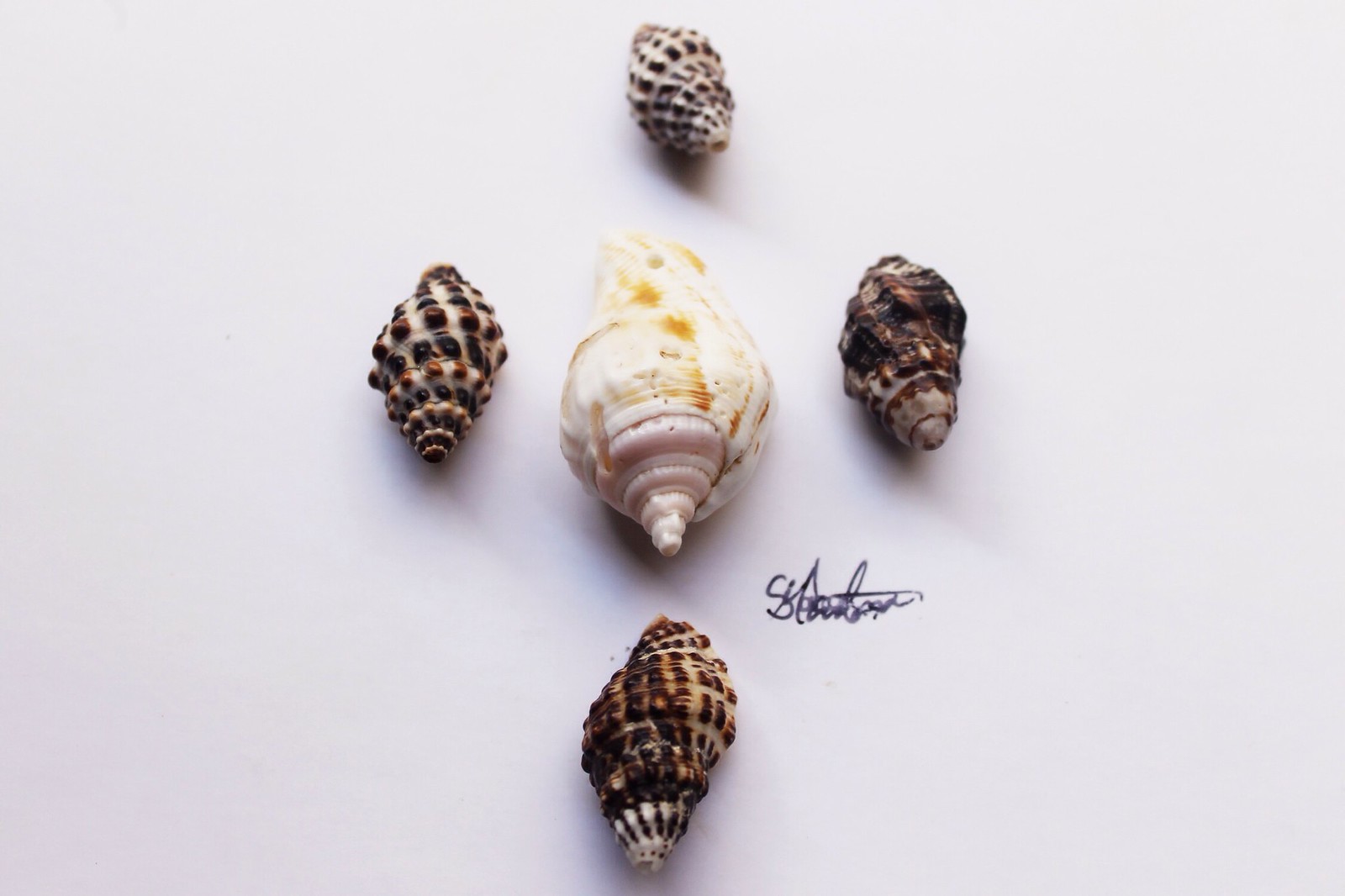The image features five seashells arranged on a white background with a gentle light casting shadows beneath them. At the center lies a large, predominantly white seashell adorned with irregular yellow marks, both circular and linear, which culminate in a spiral tip at the bottom. Surrounding this central shell are four smaller seashells positioned to its left, right, above, and below.

The three shells positioned directly above, below, and to the left of the central shell are characterized by their bumpy textures, with bumps colored in shades of brown, black, and yellow, and they all taper to a circular point at their ends. The seashell to the right of the central one differs in texture, featuring pronounced grooves that create a wavy, ribbed appearance, and it also ends in a pointed tip. The grooves, primarily black or dark brown, distinctly contrast the white base of the shell.

Between the middle-right and bottom seashells, there is a visible signature inscribed in black ink on the white background. This signature adds a personalized element to the composition, standing out amidst the shadowed areas beneath the shells.